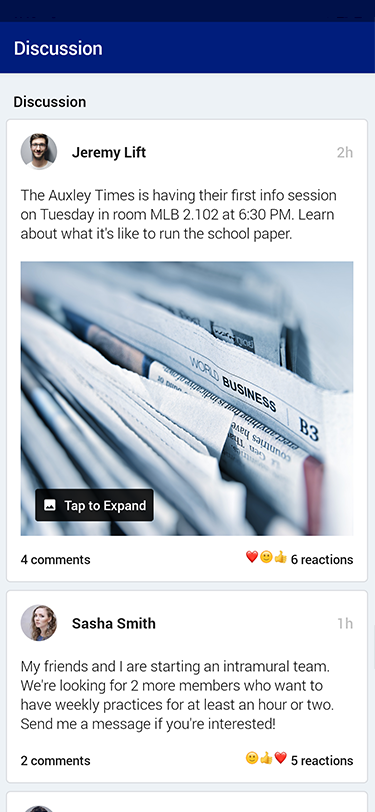This image is a screenshot depicting a discussion page, reminiscent of Facebook's interface with a mix of white and gray tones. At the top, a dark blue banner titles the page "Discussion."

The first post, authored by Jeremy Lift two hours ago, announces an upcoming event: "The Oxley Times is having their first info session on Tuesday in room MLB 2.102 at 6:30 p.m. Learn about what it's like to run the school paper." Accompanying this text is an image of stacked newspapers. The post has garnered four comments and six reactions, including hearts, smiling faces, and thumbs up.

Below Jeremy's post, Sasha Smith shares her own update from one hour ago: "My friends and I are starting an intramural team. We're looking for two more members who want to have weekly practices for at least an hour or two. Send me a message if you're interested." Her announcement has received two comments and five reactions, mostly consisting of smiley faces, thumbs up, and hearts.

The layout and interaction tools suggest this could be a form of social media or a meetup page dedicated to facilitating discussions and events.